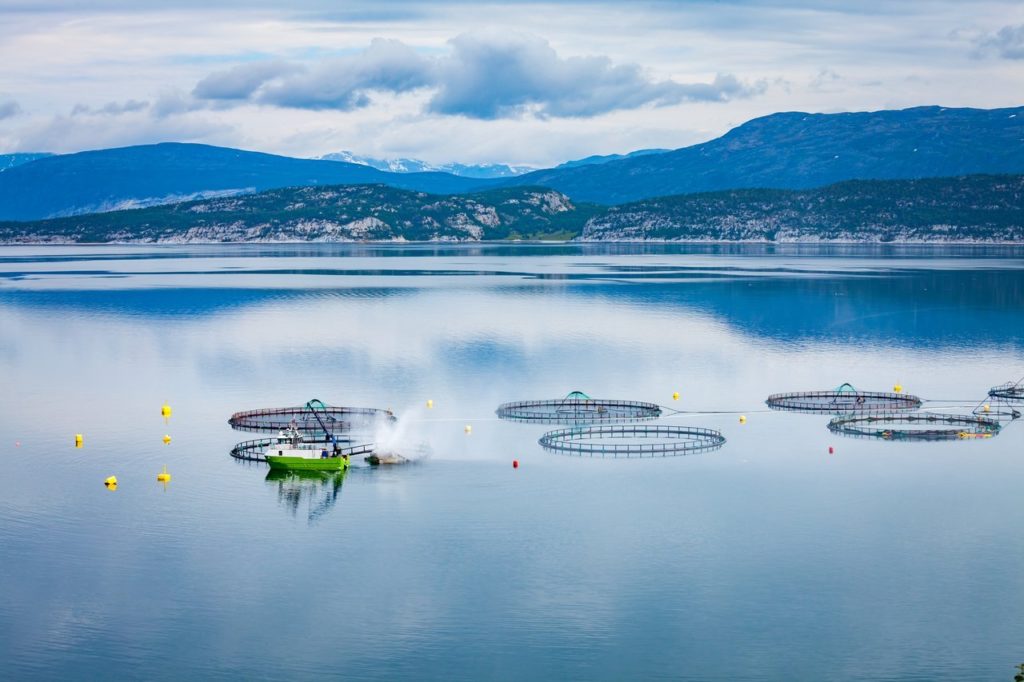This photograph captures a serene yet industrious fishing operation set against a dramatic natural backdrop. In the foreground of the blue body of water, there are multiple round fish enclosures, predominantly green, with one distinct red enclosure at the top left. These wire-enclosed, circular nets are accompanied by a collection of bright yellow, red, and orange buoys, with ropes interconnecting them. A green and white boat, stationed near the bottom left enclosure, features a large crane extending from its stern, possibly used for managing the nets. A worker on the boat appears to be engaged in operational tasks. Behind this lively scene, rolling mountains rise, their closer slopes lush with green foliage, gradually yielding to snowy caps in the distance. Overhead, a light blue sky interspersed with dark grey clouds lends an overcast atmosphere to the scenic vista. The mountains and cloud reflections enhance the tranquil ambiance of this outdoor setting, melding industry with nature seamlessly.